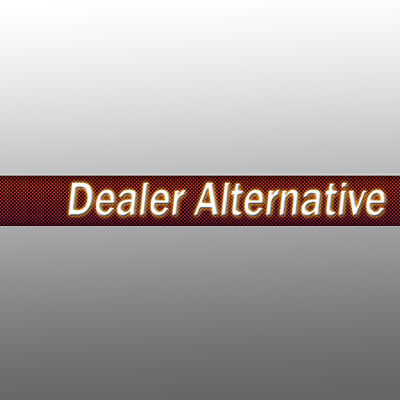The image features a minimalist design with a smooth gradient background that transitions from white at the top to dark gray at the bottom. Dominating the center of the image is a horizontally-aligned red banner that stretches from the left side to the right. This banner has a slight checkered pattern comprised of very small diamond-like shapes in black and white. Inside the banner, in large, bold white text with a red border, are the words "Dealer Alternative." The text stands out prominently and is centrally placed within the banner. The only deviation in color within this simple yet striking composition is the red banner with its text, drawing immediate focus to the words "Dealer Alternative" against the otherwise monochromatic gradient background.